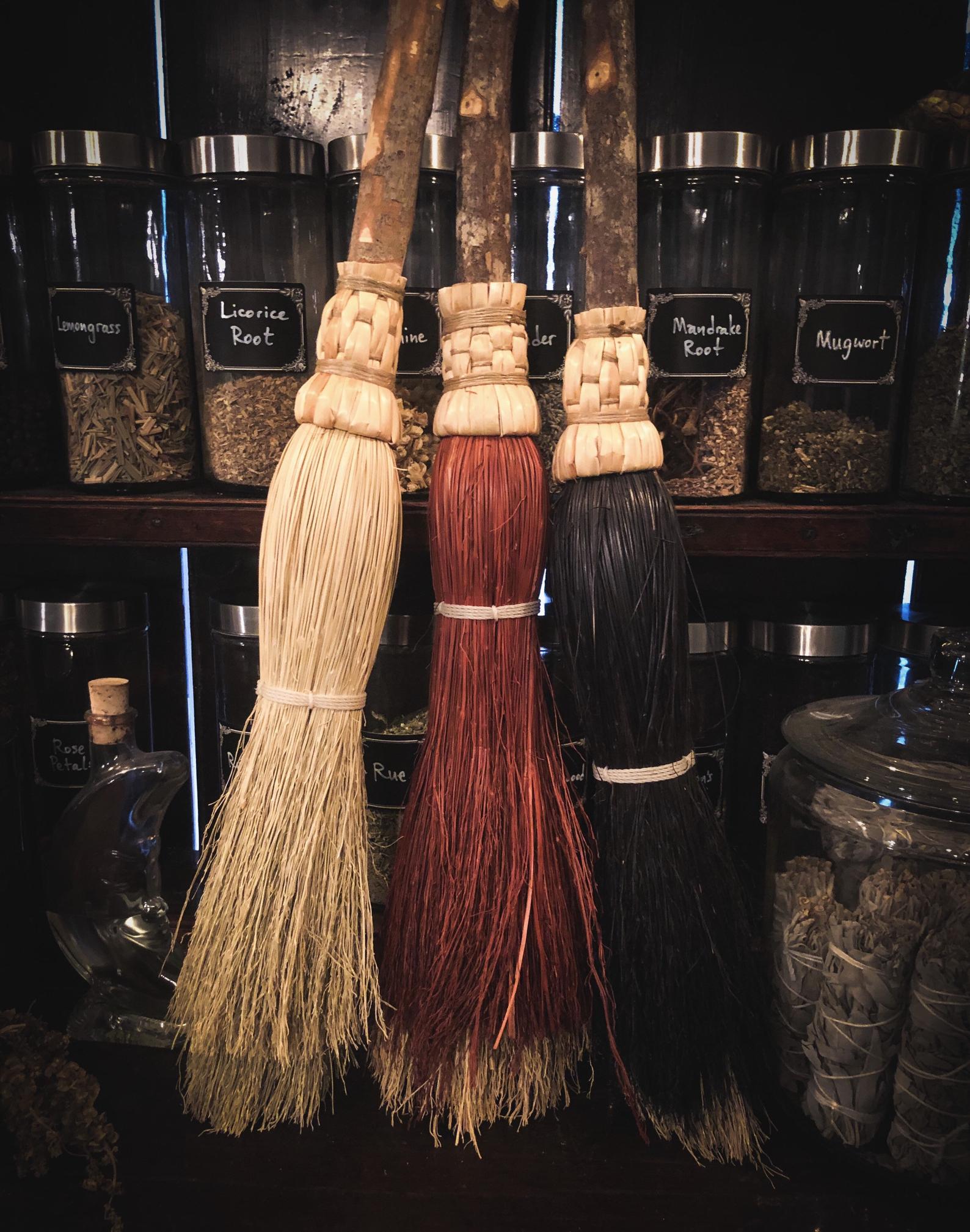The photograph depicts a rustic scene likely from a pagan or Wiccan shop featuring three homemade brooms hanging in front of a wooden shelf filled with various herbs. The brooms are crafted with unshaven sticks and differ in straw color: one beige, one red, and one black. Behind the brooms, tall cylindrical glass jars with silver tops are neatly arranged on the shelf, labeled with black labels and white writing indicating their contents. Visible herbs include lemongrass, licorice root, mandrake root, mugwort, rose petal, rue, and sage. Each jar varies in fullness, ranging from a quarter to half filled. The shelf itself is set against a brown wall, adding to the earthy, natural vibe of the space. Off to the far left is a distinctive glass bottle shaped like a quarter moon with a cork top, possibly empty, adding to the mystical ambiance. This photograph likely captures a scene from an herb shop or a witch's personal collection of magical ingredients used for rituals and spellcasting.